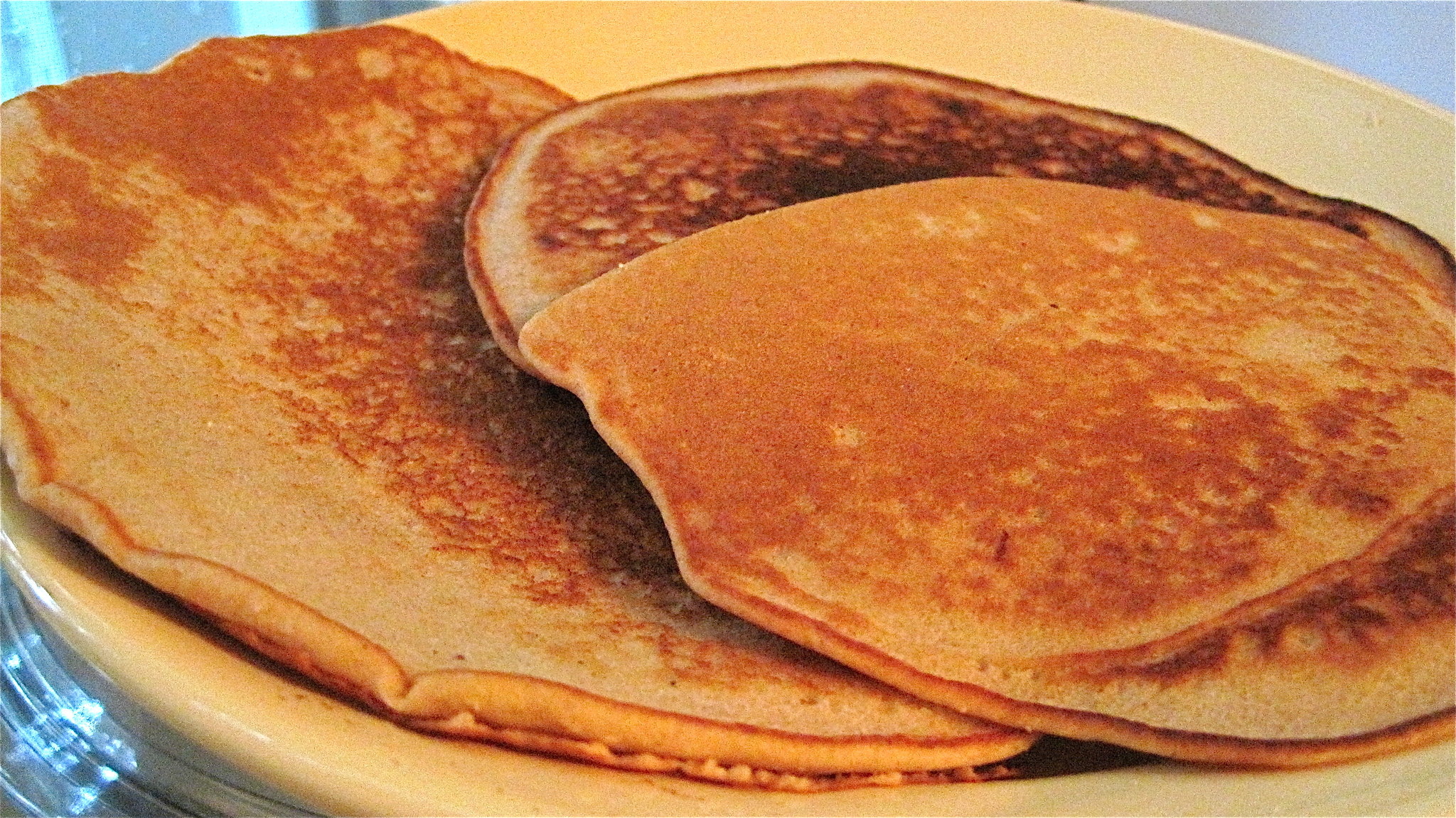This detailed photograph features three circular pancakes arranged on a round plate. The plate, which appears to be a pale yellow or off-orange ceramic, is positioned on a reflective surface, likely a clear glass table with a silvery, dark blue tint visible in the corners of the image. 

The three pancakes exhibit varying degrees of doneness. The large pancake on the lower left appears to have a nice golden-brown hue, indicative of proper cooking. In contrast, the pancake in the center stands out with its noticeably burnt appearance; its center is almost black, surrounded by an overly white ring, suggesting it was overcooked. The third pancake, to the right and slightly above the others, returns to a more uniform golden-brown coloring, similar to the first, ensuring that the outer pancakes appear properly cooked while the middle one is visibly overdone.

No toppings such as butter or syrup adorn these pancakes; they are served plain, with their textures and colors telling their own story without the embellishment of condiments.